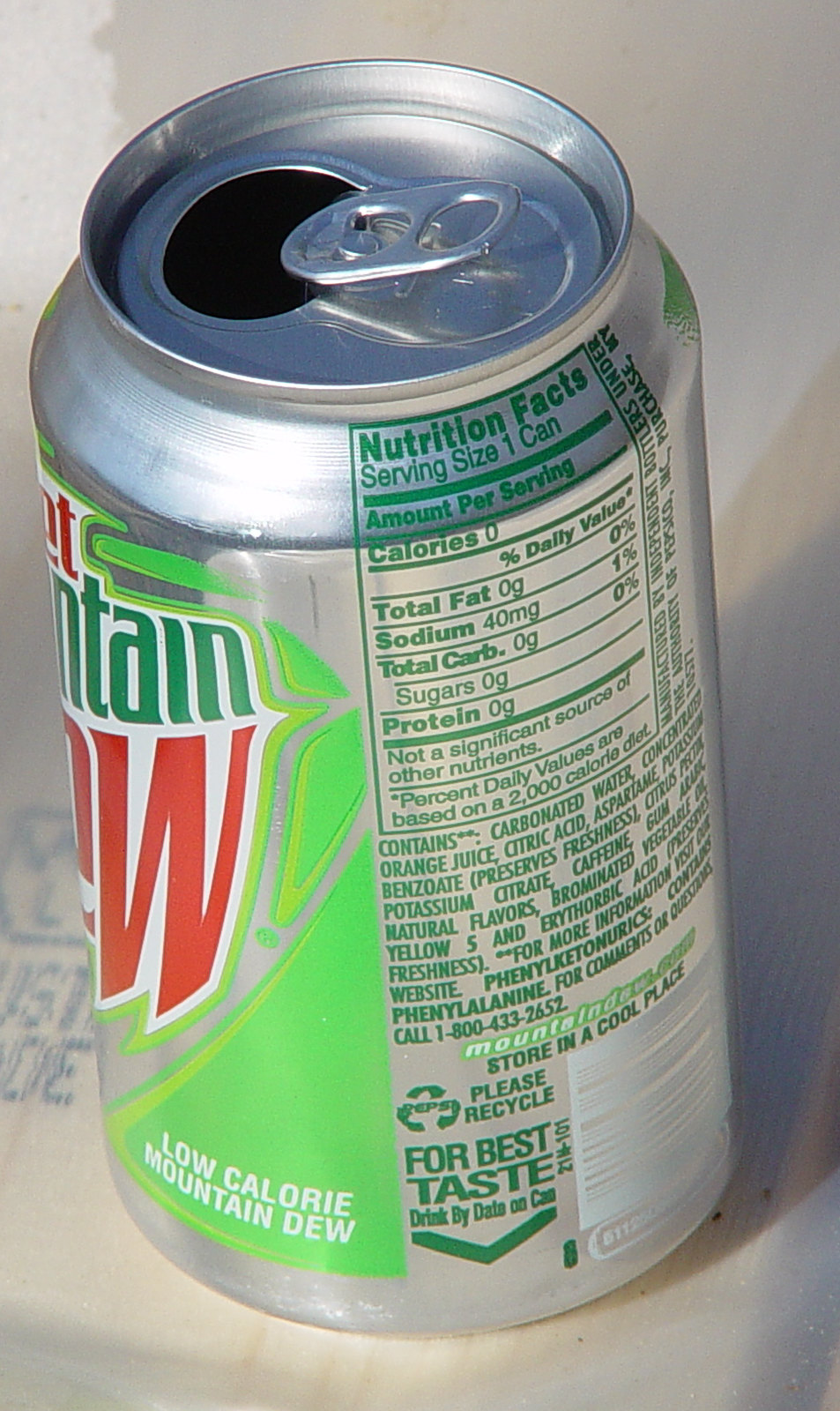The photograph depicts a partially opened aluminum can of Diet Mountain Dew placed against a white background, likely on a desktop or table. The can features the iconic silver coloring with green, red, and white logos. Prominent on the can is the Diet Mountain Dew branding, with the word "Diet" partially visible above "Mountain Dew." The can is turned about 45 degrees to the left, revealing the nutritional information in green. This data includes a serving size of one can, zero calories, zero total fat, 40 milligrams of sodium, zero carbohydrates, zero sugars, and zero proteins, along with the note that it is not a significant source of other nutrients. The can lists ingredients such as carbonated water and includes a recycling logo with the instruction to "store in a cool place, please recycle," and "for best taste, drink by the date on the can." Additionally, there is a white UPC code on the silver surface and some illegible print in the bottom left, which appears to resemble a blueprint.